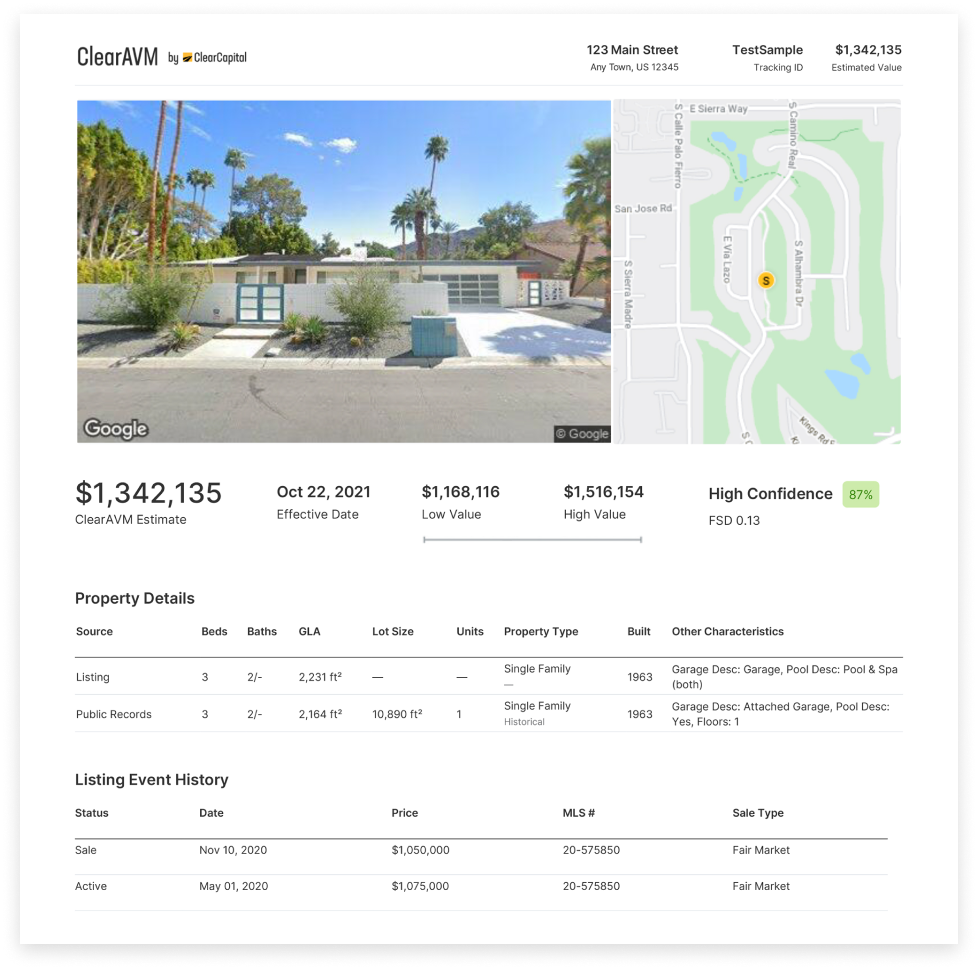A screenshot from the ClearAVM website, developed by ClearCapital, features prominently at the top of the page with its name. To the right, there's an address listed as "123 Main Street, Anytown, U.S. 12345." Beneath the address, there's a label indicating "test sample" and an adjacent estimated property value. 

The central part of the page displays an image of a white ranch house with blue trim. The house has a garage and a blue gate at the front, surrounded by palm trees and other desert vegetation indicative of an arid climate. Next to the house image, there is an overhead map view pinpointing the property's location. The estimated value of the house, as shown on the webpage, is $1,003,042.13.